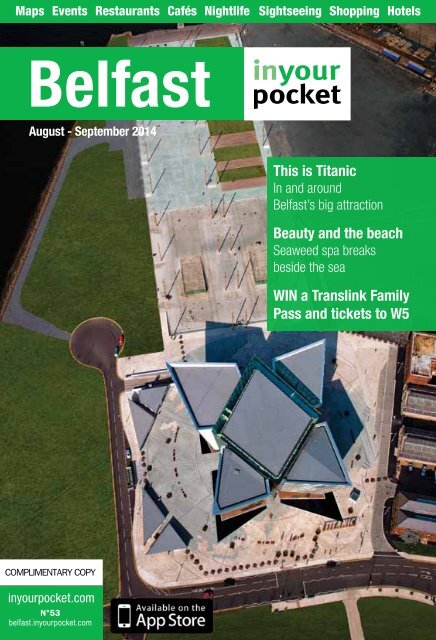The magazine cover titled "Belfast In Your Pocket" features an aerial photograph of the modern and architecturally striking Titanic Belfast building. The cover has a green band at the top with white text listing categories including maps, events, restaurants, cafes, nightlife, sightseeing, shopping, and hotels. Positioned beneath this band, the words "Belfast In Your Pocket" are prominently displayed above another green strip indicating the publication date, August to September 2014. The main visual element is the Titanic Belfast, described as a significant attraction in the city. The structure is highlighted with accompanying text, "This is Titanic in and around Belfast's big attraction," suggesting its importance. The photograph shows the building's intricate design, which appears to consist of a central diamond-shaped section flanked by five other geometric, possibly pentagon-shaped, segments. This guide aims to provide tourists with essential information and insights about Belfast’s attractions and amenities.